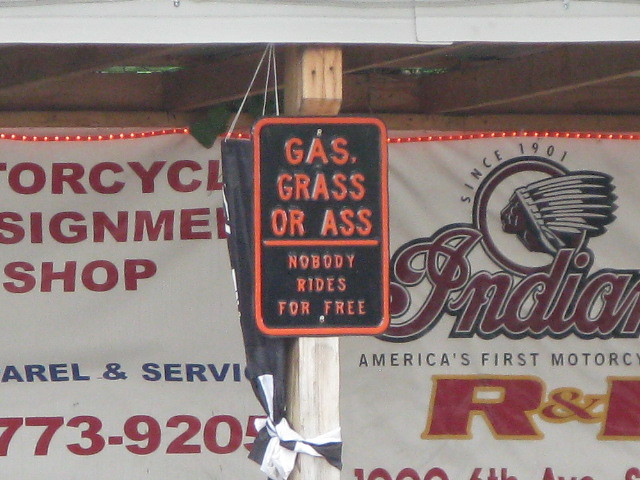In this detailed photograph, we are at an event setting featuring a variety of signs attached to a wooden post wrapped in a black and white banner, situated under light-colored wooden rafters. Prominently displayed at the center is a vertically-oriented rectangular sign with a black background and an orange border, bearing the memorable imprinted phrase in capitalized text: "GAS, GRASS, OR ASS, NOBODY RIDES FOR FREE."

To the left-hand side of the image, there is a partially visible banner displaying red text on a white background. It appears to belong to a motorcycle shop, though some of the words are cut off, it includes fragments like "O-R-C-Y-C-L," "S-I-G-N-E-M-E," "shop," "apparel and service," and a phone number, "773-9205."

On the right-hand side, another banner hangs, also in red on white, proclaiming "Indian, America's first motorcycle since 1901" alongside a red image of a Native American in a headdress. The banner includes the phrase "R &" before being cut off at the edge of the image. This vivid and eclectic assortment of signage creates a visually striking scene that captures the atmosphere of the event.